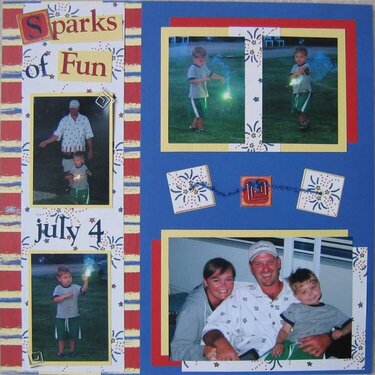The image appears to be the front of a personalized scrapbook or poster made of various photographs and colorful decorations. It features a collage of five different personal family photos, each showcasing moments from a July 4th celebration. The primary colors used in the design are red, white, blue, yellow, gray, and green, giving it a festive and patriotic appearance. At the top, the text "Sparks of Fun July 4th" is prominently displayed, accented with a decorative vertical banner on the side that includes a pattern of red, blue, and yellow lines.

The photos are arranged in a slightly random but harmonious manner, emphasizing the scrapbook style. The images capture various moments: one shows a man and a young child holding a sparkler, another features a small boy with a sparkler glowing bright and emitting smoke, and additional photos in the top right corner depict the boy holding the sparkler in different poses. At the bottom, a family portrait showcases a woman on the left, a man in a baseball cap in the center, and a smiling child in a gray shirt and green shorts on the right. The overall composition is lively and nostalgic, celebrating family and festive moments.